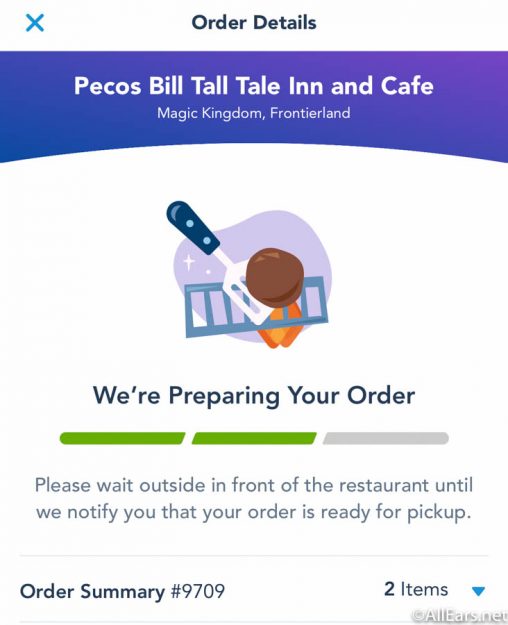This vertical rectangular image features a clean, organized design conveying order details. At the very top, a white border presents a blue "X" icon on the far left, with 'Order Details' centrally written in black text. Below this, a semi-curved banner with a purplish-blue hue hosts white text reading 'Pecos Bill Tall Tale Inn and Café, Magic Kingdom, Frontierland.’ 

Underneath this banner, there is an illustration of a spatula holding what appears to be a hamburger patty, accompanied by grill marks. An orange, square-like element is also included in this section. The background of the main section is white, and directly beneath the spatula and patty, there is bold text in dark blue or black declaring, 'We're preparing your order.'

Below this message, a status progress bar is segmented into three parts—two of which are highlighted in green, indicating progress, while the third segment is grayed out. Additional instructions advise, 'Please wait outside in front of the restaurant until we notify you that your order is ready for pickup.' At the very bottom, in black text, it states 'Order Summary 9709, 2 items.'